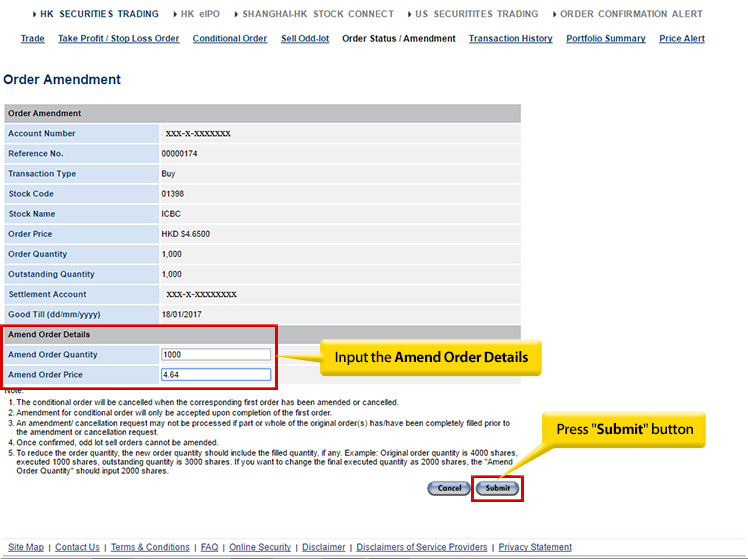The website interface for HK Securities Trading is displayed, featuring key options like "HK EIPO," "Shanghai HK Stock Connect," "U.S. Securities Trading," and "Order Confirmation Alert." Below these options is a menu that includes various trading actions: "Trade," "Take Profit," "Stop Loss Order," "Conditional Order," "Sell," "Odd Lot," "Order Status," and "Amendment," with the latter being currently selected. Further options available are "Transaction History" and "Portfolio Summary."

In large blue text, the page highlights "Order Amendment." A grey header displaying the same text is positioned below. On the left side of the screen, numerous blue text buttons, which might be clickable, list several account details: "Account Number," "Reference Number," "Transaction Type," "Stock Code," "Stock Name," "Order Price," "Order Quantity," "Outstanding Quantity," "Settlement Account," and "Good Till."

To the right, several "X" icons are visible alongside detailed transaction data: Account Number 174, Buy order for Stock Code 1398 (ICBC), priced at HKD $4.65, with an Order Quantity of 1000 and an Outstanding Quantity of 1000. The "Good Till" date is set to 18-01-2017.

Below these details, on a grey bar, the "Amend Order Details" section allows for modifying the quantity and order price, which is entered as $1004.64. Highlighted in a red rectangle is a yellow speech bubble instructing users to "Input the Amend Order Details." Further down, text within another red rectangle, accompanied by a yellow speech bubble, directs to "Press Submit button," positioned near the "Cancel" and "Submit" options. The page footer includes links for the "Sitemap," "Contact Us," and "Terms and Conditions."